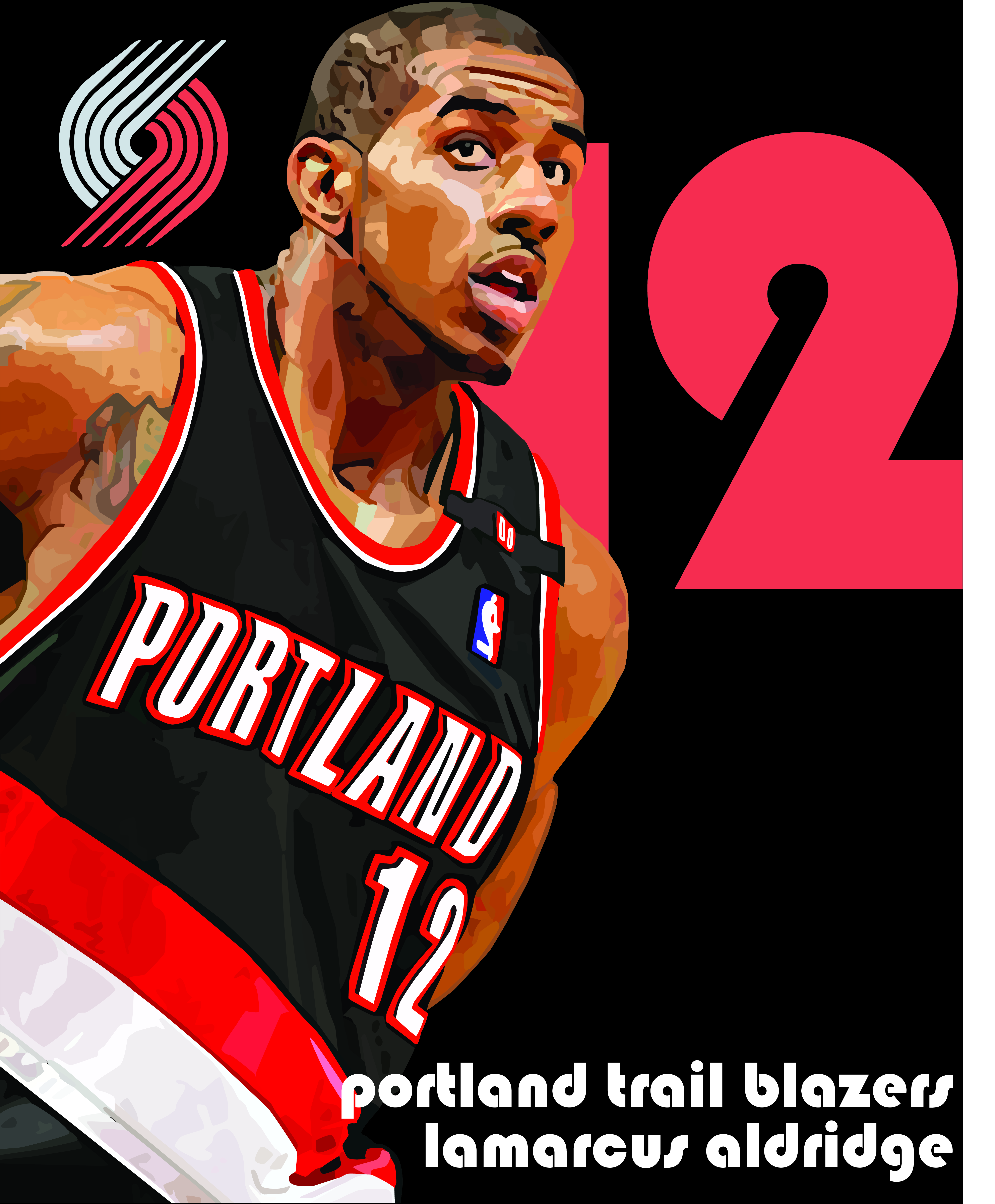In this promotional posterized press photo, we see African American basketball player LaMarcus Aldridge, captured in a dynamic, abstract style. Posed at an incline from the bottom left to the top middle of the image, Aldridge's intense expression features an open mouth, slightly revealing his top teeth and tongue, and a well-groomed mustache. He sports a black Portland Trail Blazers jersey, distinctively adorned with red and white stripes across the middle and matching trim around the collar and sleeve area. The jersey bears the white text "Portland 12" prominently across his chest, with the official NBA logo on his left side. Peeking just above the neckline of his jersey is a visible tattoo near his shoulder.

The backdrop is primarily black, against which vibrant elements are juxtaposed—on the top left, a red and gray swirling logo, and towards the upper right, a large, blocky number "12" in retro-style red font. The text, "Portland Trail Blazers LaMarcus Aldridge," is superimposed at the bottom right, further emphasizing the promotional nature of this striking image.